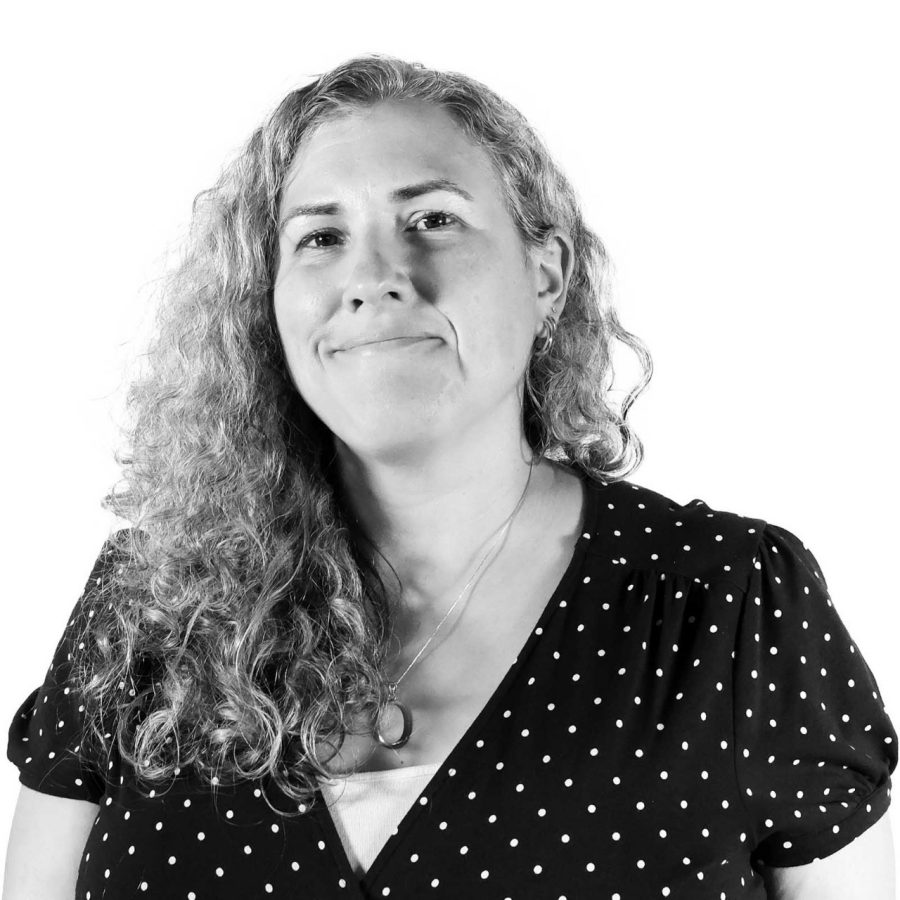The monochrome portrait captures a woman of light complexion, likely in her late 30s to mid-40s, against a stark white background. With wavy, slightly frizzy hair falling to her chest, her hairstyle hints at blonde tones. She gazes directly at the camera with her lips pressed into a subtle smile, emphasizing fine lines on her cheeks. She dons a short-sleeved, dark-colored top adorned with tiny white polka dots, featuring a low-cut V-neck that reveals a part of an inner garment. Around her neck hangs a delicate gold necklace with a round hollow ring pendant. Her accessories also include three earrings—two hoops and a stud in her right ear—and the overall setting is brightly lit, ensuring clarity and detail in the image.